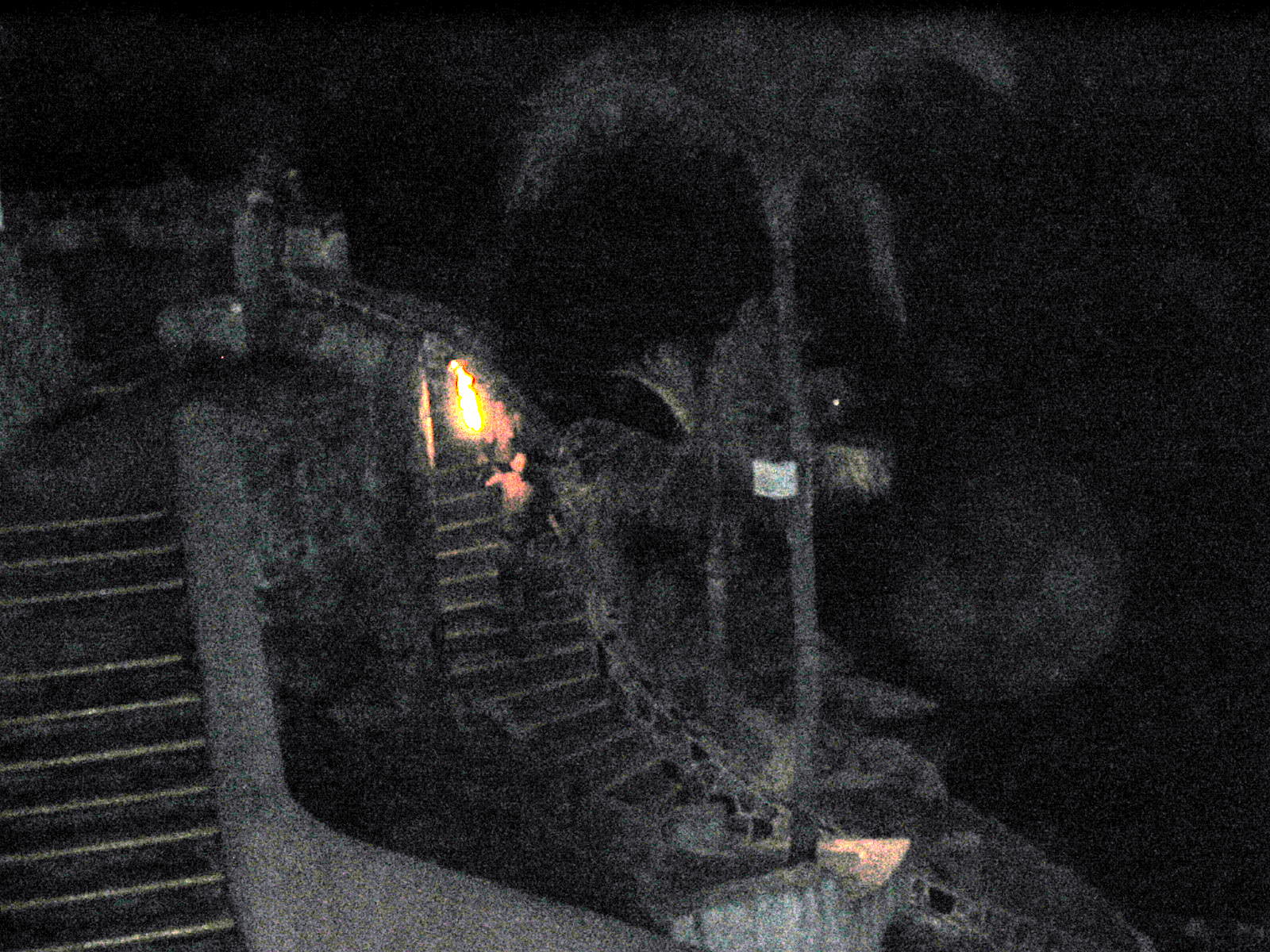In the darkness of night, a solitary figure ascends an outdoor staircase adjacent to a building, seemingly in the act of lighting a flame or possibly firing a gun. The flame, potentially emanating from a lantern, casts a vivid red glow that envelops the person's form, standing out starkly against the otherwise monochromatic backdrop. The scene is cloaked in shadows, giving it a nearly black-and-white appearance. Amidst the dimly lit surroundings, silhouettes of palm trees and additional steps are discernible. At the top of the staircase, there is a faint glimpse of another person holding a white lamp, contributing to the mysterious ambiance. The eye is irresistibly drawn to the central flame, which appears intimately connected with the actions of the ascending figure, creating a captivating focal point in the image.